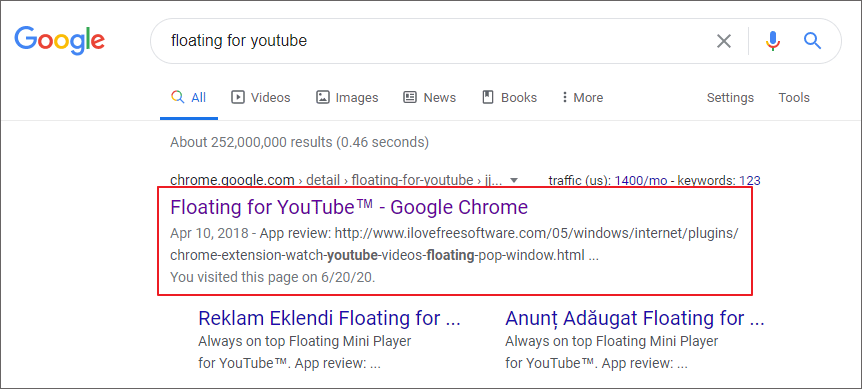This image captures a Google search results page. At the top left corner, the Google logo is visible. In the search bar, the query "floating for YouTube" is entered. Below the search bar, search results are displayed. A red box highlights the first search result titled "Floating for YouTube™ - Google Chrome" dated April 10, 2018, described as an app review. The URL provided is "www.ilovefreesoftware.com/05/windows/internet/plugins." An additional line indicates that this is a Chrome extension for watching YouTube videos in a floating pop-up window, with the specific address "watch-youtube-videos-floating-pop-window.html." It also notes that the page was visited on June 2020.